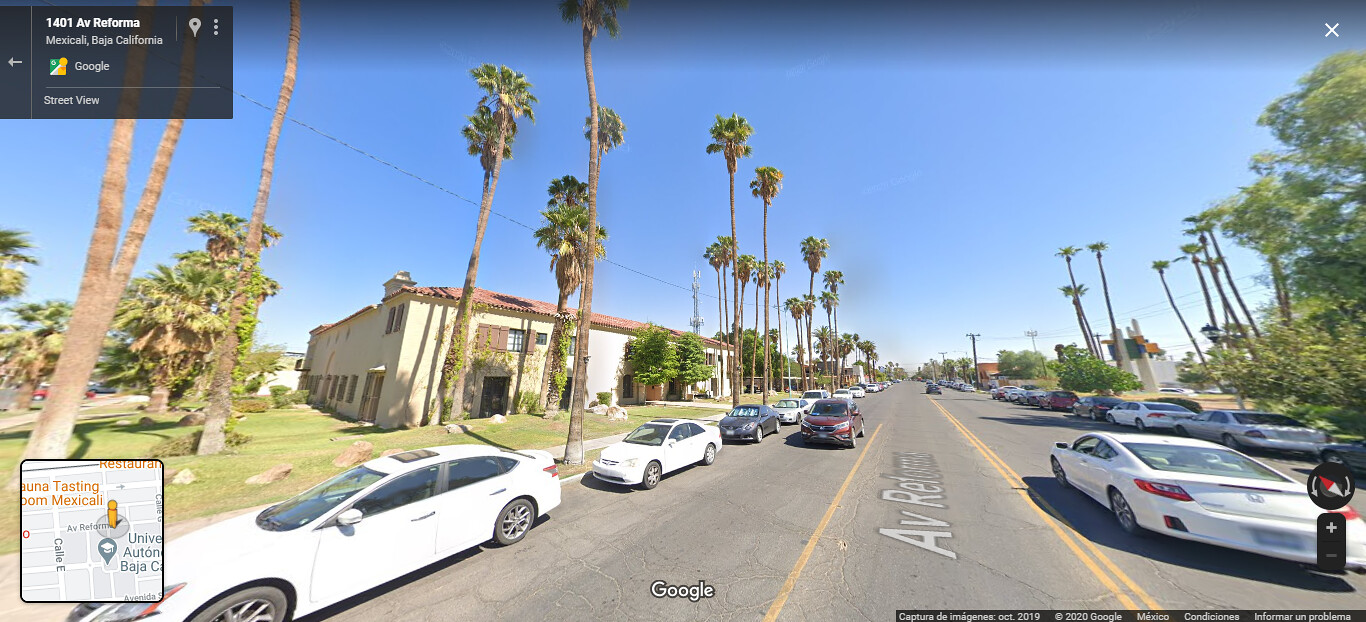The image depicts a Google Street View scene featuring a sunlit, palm tree-lined street, likely located on the west coast of the United States, specifically California, as indicated by the address details in the top left corner of the screenshot. The scene is captured with a fisheye lens effect, resulting in a wide field of view that stretches and distorts the appearance of the cars on the road. This screenshot, taken on a computer, displays the typical Google watermark at the bottom right corner, confirming its origin. The address appears to be partially visible, though the precise street name is difficult to discern due to pixelation and blurriness. The bright, cloudless sky underscores the sunny Californian climate, contributing to the overall vibrant and warm atmosphere of the captured street view.